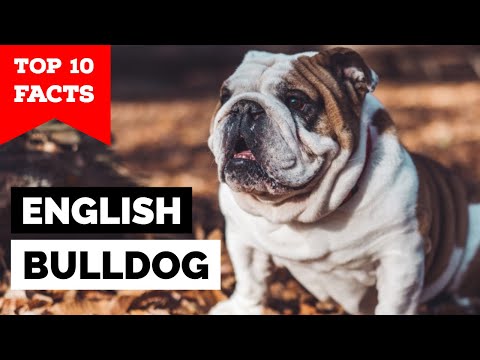This image showcases a charming English Bulldog in a backyard setting. The Bulldog, standing on some grass with scattered dried leaves, is white with distinctive brown spots, particularly around its eyes and on its body. The dog has a black nose and a partially open mouth, revealing its bottom teeth. Its gaze is directed forward, and the shadowing from overhead trees adds depth to the grassy background.

The photograph is framed with black borders at the top and bottom. In the upper left corner, there's a red banner with a triangular cutout at the bottom. The banner features the text "Top 10 FACTS" in bold, capitalized white font, split across two lines. Directly below this are two rectangles: the first is black with the word "ENGLISH" in white capital letters, and the second is white with the word "BULLDOG" in black capital letters. The overall scene highlights the Bulldog’s endearing features amidst a subtly detailed outdoor backdrop.